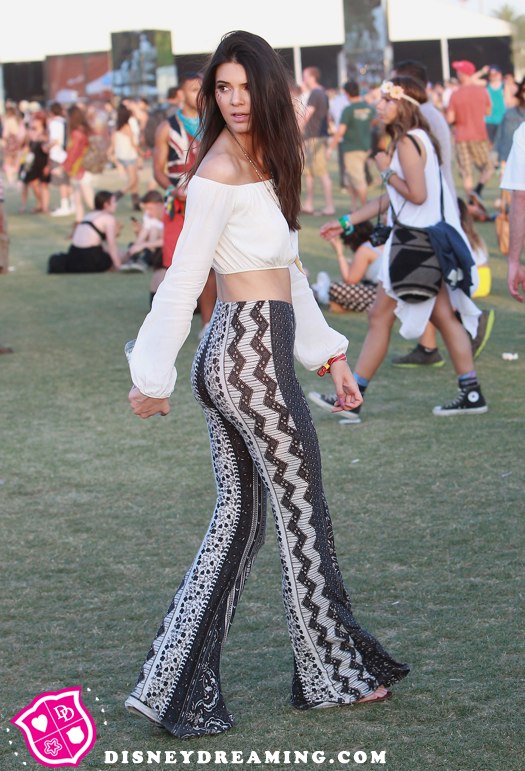This photograph, taken by DisneyDreaming.com, features a woman who is the main subject of the image. She has long, dark brown hair that falls to her chest and is wearing an off-the-shoulder white crop top with long, elasticated sleeves. Her ribcage is slightly visible. She pairs the top with distinctive, bell-bottom pants that showcase a black, white, and darker brown squiggly design, and she completes her look with sandals and a gold necklace. The woman is captured in a walking position, with her body facing right but her head turned back to look over her left shoulder. The background is a grassy park area with various people moving about, dressed in a range of colors including white, green, brown, yellow, beige, blue, and black. Notably, one person in the crowd is clad in a shirt featuring the British flag. The bottom of the image includes the DisneyDreaming.com website address in white text, superimposed on the grass. Additionally, there is a pink shield logo on the bottom left, divided into four quadrants: a heart in the top left, two intertwined Ds in the top right, a five-pointed star in the bottom left, and another white shield in the bottom right, all separated by a white cross.